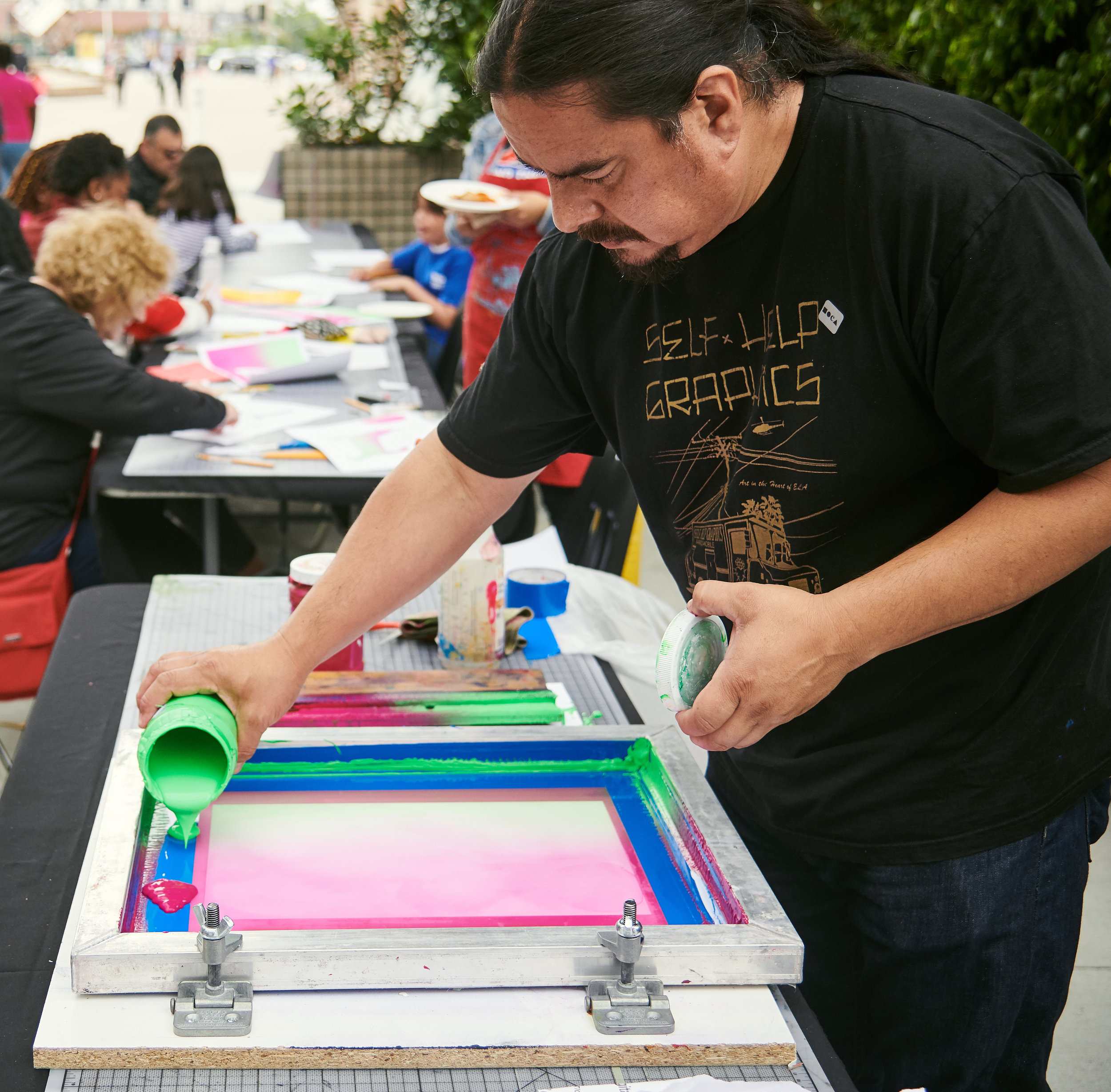This color photograph captures a man engaged in the process of screen printing. Positioned to the right of the frame, he stands beside a table on his left, with additional tables and individuals working in the background. At his table, a wooden frame is set up, and he is meticulously pouring green paint from a jar into the frame, which also contains pink and blue paint. The frame is secured with two clamps visible in the foreground. The man’s distinctive black hair is tied back in a ponytail, and he is wearing a black t-shirt displaying the text "Self-Help Graphics" along with a graphic below it. The table's surface is black, adding contrast to the vibrant paints. In the background, green bushes and a street can be seen in the distance, adding depth to the scene.